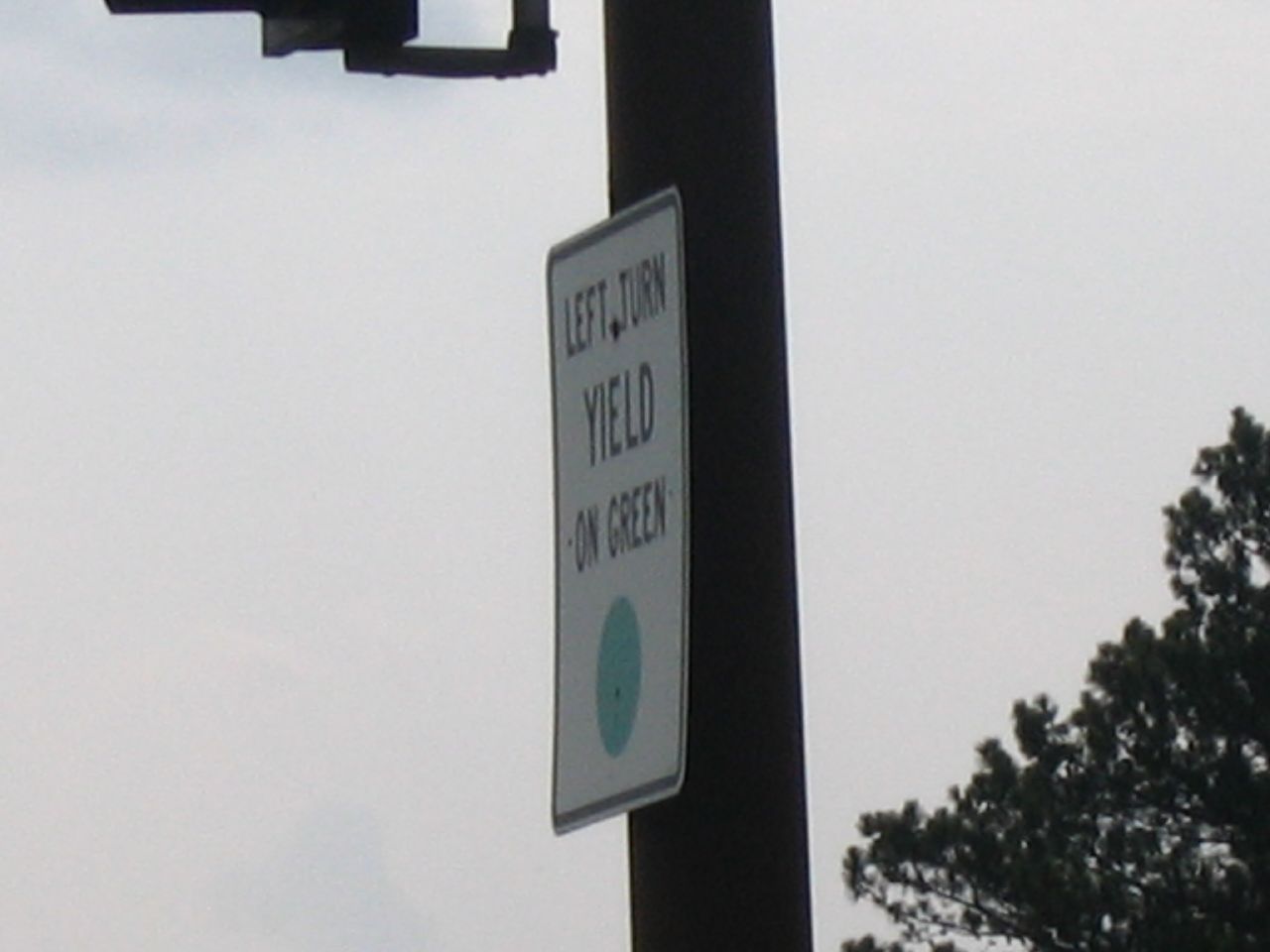The image captures a slightly blurry photograph of a white street sign affixed to a dark gray post. The sign, outlined with a black border, bears the black, all-caps inscription "LEFT TURN YIELD ON GREEN" with a green circle at the bottom. The cloudy sky in the background appears soft and gray, lacking definition or any hints of blue. A portion of a stoplight's metal structure is visible at the top edge of the photo, though no lights are discernible. Additionally, a tree with bare branches and dark foliage is situated in the background, adding to the moody, overcast atmosphere captured in the scene. No cars or additional signs are present in the photograph, focusing attention solely on the sign, the overhanging stoplight structure, and the solitary tree.